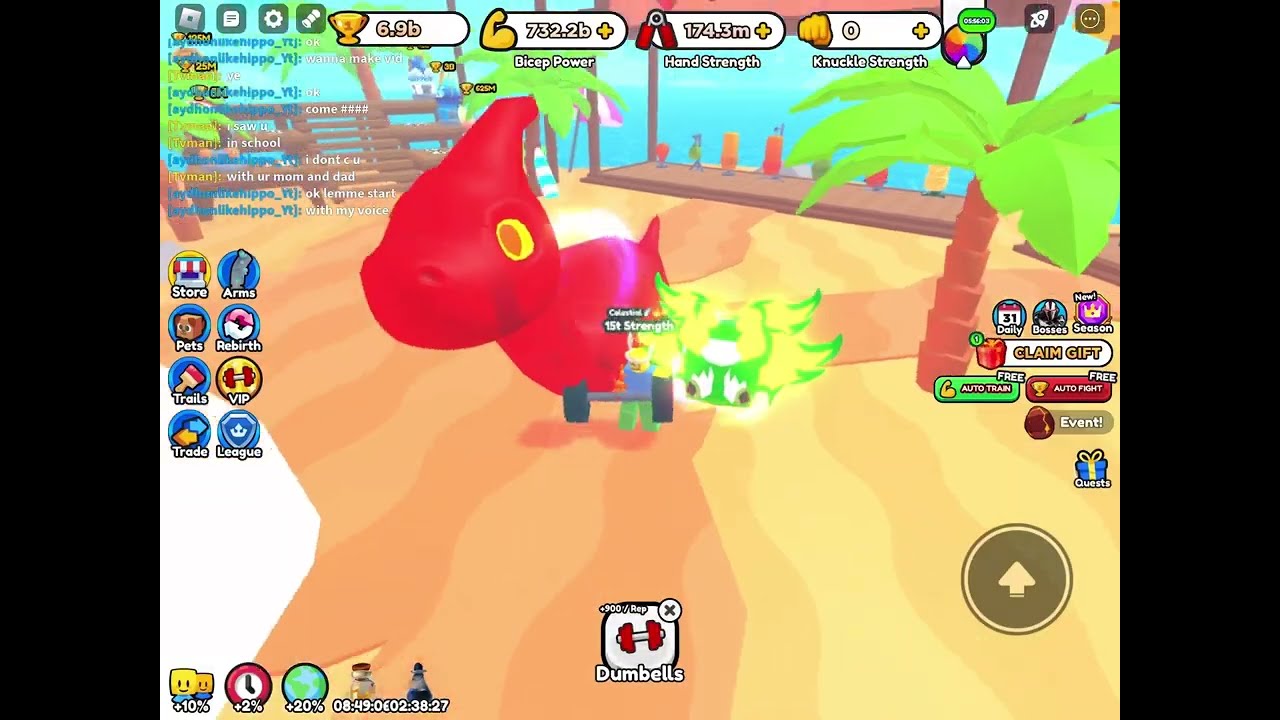This vivid screenshot from an unidentified video game captures a bustling beach setting with a central Lego-style character lifting a red dumbbell. The character, with yellow skin, a blue shirt, and green pants, stands on beige sand, framed by diverse elements. To his left is a large red horse-like creature on black wheels with yellow eyes and red pupils. To his right, a green and white flying creature with front-facing eyes hovers, while a lush palm tree with a brown trunk and green leaves stands nearby. In the background, the serene ocean stretches out, bordered by wooden stands and onlookers. The game interface is filled with various controls and information, including displays of numbers and rewards like 6.9B and 732.2 at the top, alongside function labels such as Store, Arms, Pets, Rebirth, Trails, VIP, Trade, League with corresponding logos on the left. The bottom of the screen features a red dumbbell icon with white text reading "Dumbbells," and there's a navigation arrow on the right. Additional labels for "claim gift," "auto-train," "auto-fight event," and "guests" populate the screen, contributing to a dynamic and interactive gaming experience.